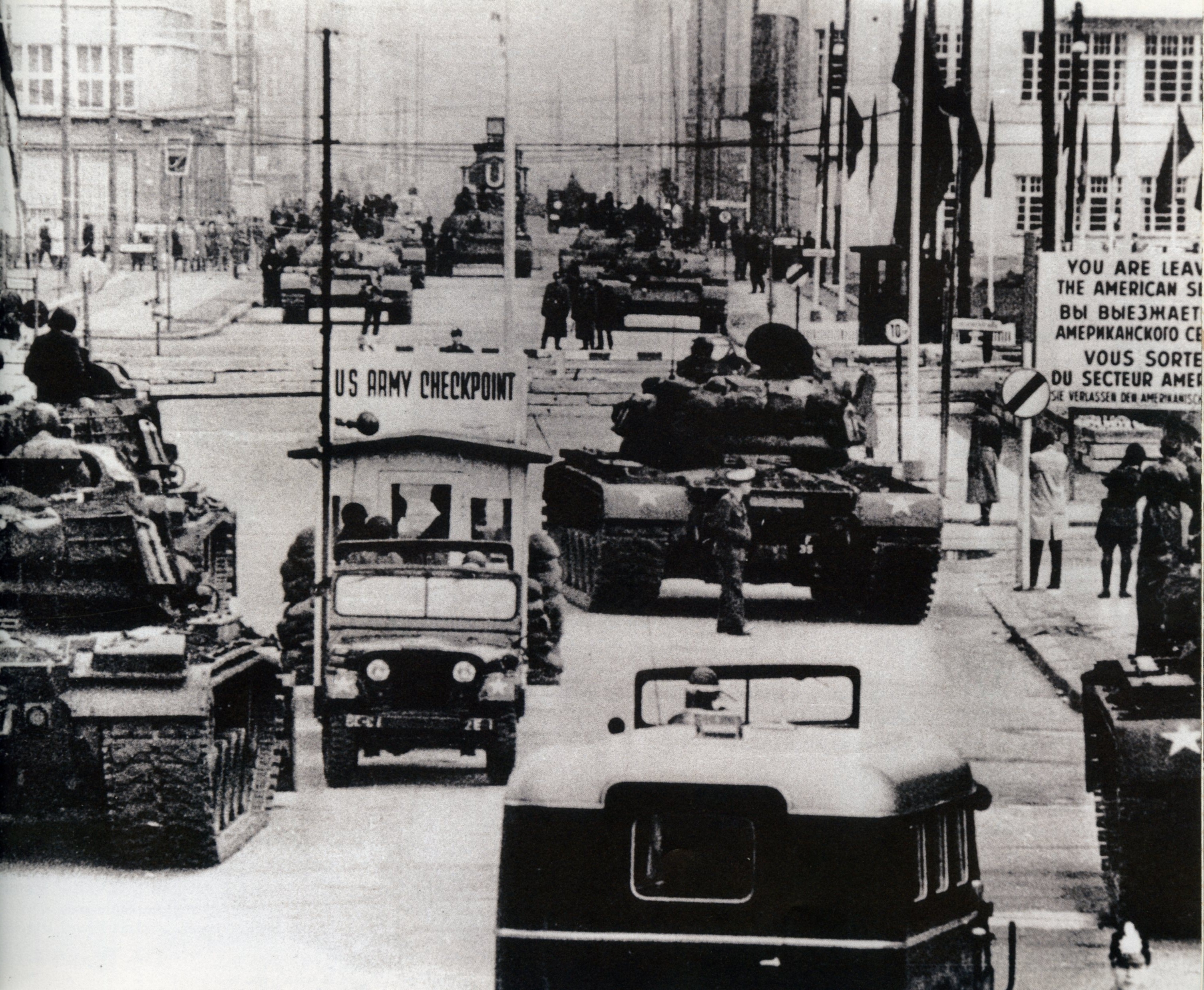This detailed black and white vintage photograph captures a bustling city street scene that appears to be from World War II in Europe. Dominating the street are numerous military vehicles, including tanks and jeeps, which are driving towards the camera. One prominent jeep features a sign above it reading "U.S. Army Checkpoint." The street is lined with tall buildings adorned with windows, and various flags can be seen lining the right side, enhancing the militaristic atmosphere. In the right-hand corner, there’s a partially visible sign with multilingual text indicating a boundary: "You are leaving the American... Vous sortez du secteur américain,” suggesting this is likely a checkpoint marking the edge of the American sector. Several civilians, in dark coats and caps, as well as men in military uniforms, stand on the sidewalks, looking on as the convoy moves through. The presence of these elements, combined with the vintage quality and attire of the individuals, firmly places this captivating image in a historical wartime context.